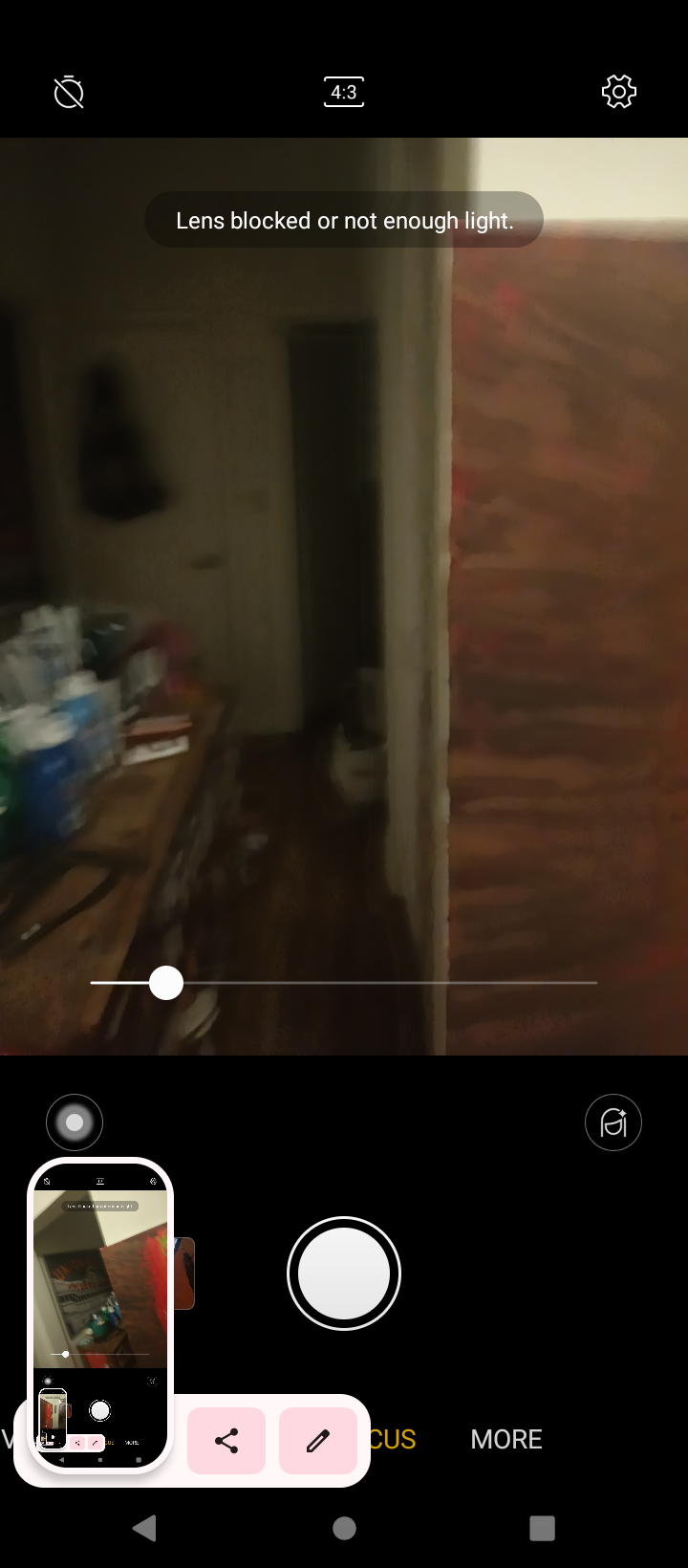This detailed image captures a screenshot of someone's phone displaying the camera app. The camera app has various symbols on top: a crossed-out stopwatch, a 4:3 ratio indicator, and a gear icon for settings. A white message at the top states, "lens blocked or not enough light." On the bottom center, there is the classic white circular button for taking pictures, flanked by additional symbols. To the lower left of the screen, previous screenshots can be seen nested within one another, creating an image-in-image effect. The actual picture being taken is blurry and depicts a hallway. The hallway features white walls, white doors with white trims, and a wood-paneled wall to the right. There is a table on the left—brown, with several indistinguishable objects, including blue containers with white caps and something black and curly. Far in the background, there is a white door with a horizontal handle, possibly with a coat hanging on its back, and an adjacent open door leading to a dark area. Below the viewfinder, there are also three classic navigation symbols for the phone: a triangle, a circle, and a square. The image captures a complex and layered snapshot of someone attempting to take a photo under challenging conditions.